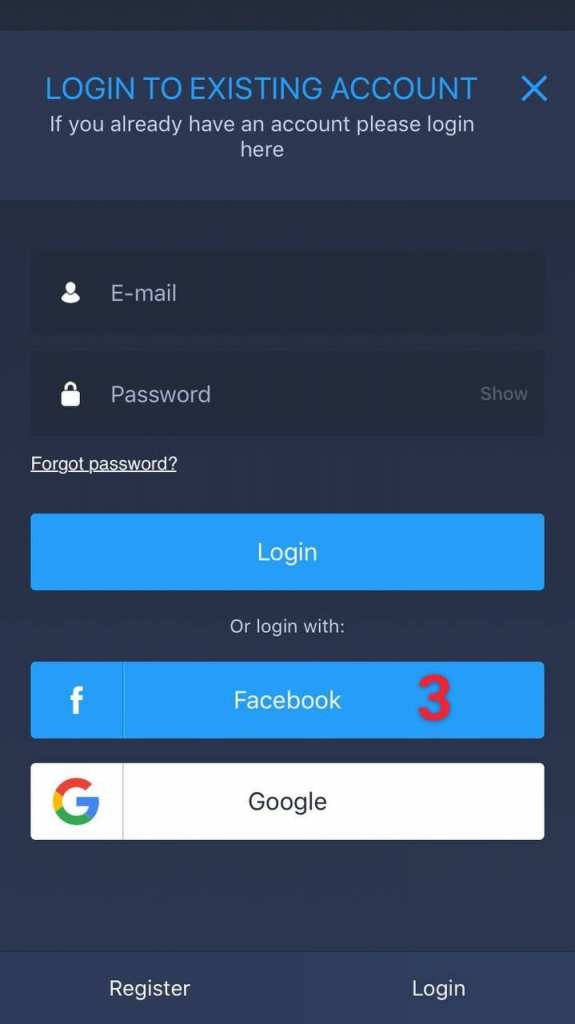A vertically oriented dark blue rectangle, almost black, dominates the image. At the top, in all capital letters and large blue font, it reads "LOG IN TO EXISTING ACCOUNT." Adjacent to this line, on the right side, there's an X icon allowing users to close this section.

Beneath this header, a white text reads: "If you already have an account, please log in here." Following this is a series of form fields. The first field, marked with a person icon on the left, has the placeholder text "Email." Below it is a second field for "Password," accompanied by a lock icon on its left. To the right of the password field, there's a "Show" option.

Under these fields, a white underlined text states "Forgot password?" for users to retrieve their credentials. 

A prominent blue button, matching the size of the form fields, displays "LOG IN" in white text. Below this button, the phrase "Or log in with:" introduces alternative login options. Two buttons of the same size as the primary login button are present. The first is blue with a white "F" for Facebook, and the second is white featuring a multi-colored "G" for Google.